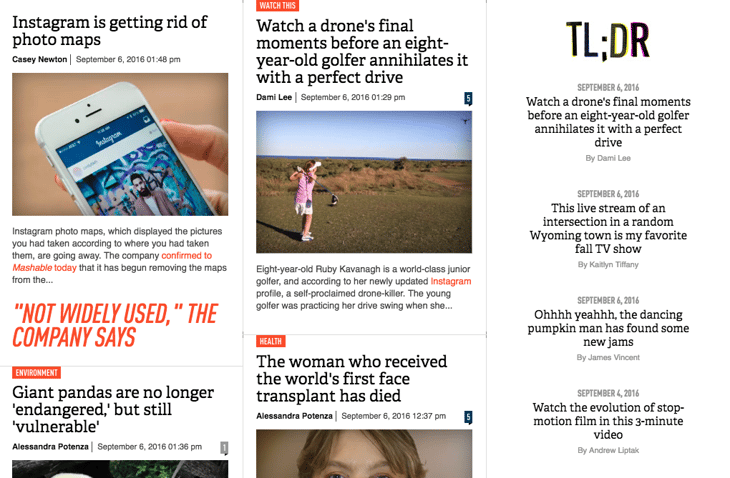**Detailed Caption:**

The image is a digitally altered screenshot depicting a website or app interface, capturing a series of news snippets and articles. In the upper left corner, there's an announcement titled "Instagram is getting rid of photo maps." Below this headline, detailed text follows: "Casey Newton, September 16, 2016, at 1:48 p.m. Instagram photo maps, which displayed the pictures you had taken according to where you had taken them, are going away. The company confirms to Mashable today that it has begun removing the maps because they are not widely used, the company says."

Adjacent to this, another headline appears: "Giant pandas are no longer endangered but still vulnerable," authored by Alessandra Potenza on September 16, 2016, at 1:36 p.m.

In the right column, there's a visually engaging story titled, "Watch a drone's final moments before an eight-year-old golfer annihilates it with a perfect drive," posted by Dami V on September 16, 2016, at 1:29 p.m. Accompanying this headline is an image of a little girl in a pink shirt, poised in a golfing stance. Below this image, the description reads: "Eight-year-old Ruby Kavanaugh is a world-class junior golfer and, according to her newly updated Instagram profile, a self-proclaimed drone killer. The young golfer was practicing her drive swing when she..."

This carefully crafted caption meticulously captures the essence and details of the content presented in the image.